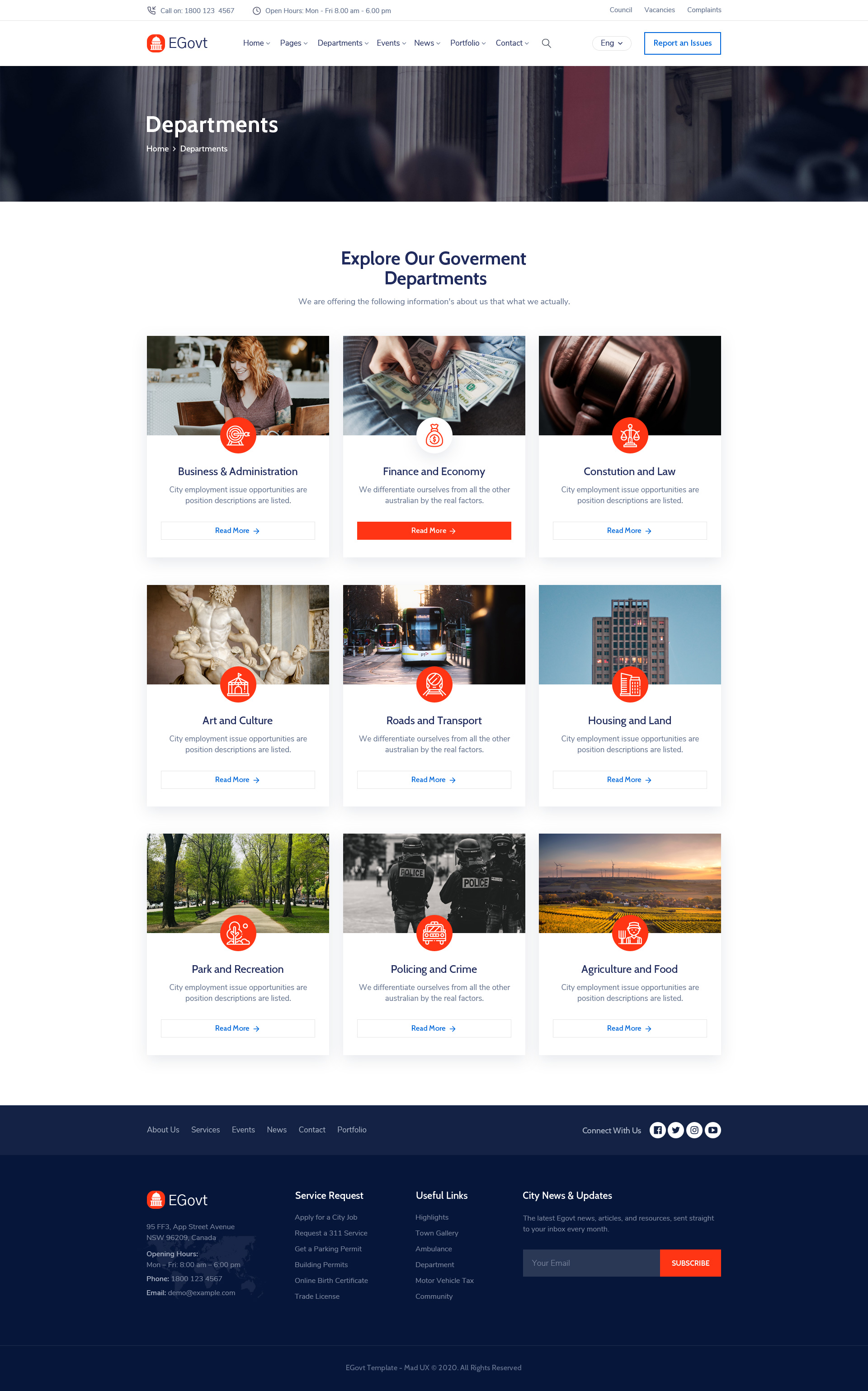Screenshot of the E-G-O-V-T Website Homepage:

At the top of the webpage, the website is branded with the label "E-G-O-V-T," accompanied by a small, indistinct icon resembling a red square with white lines beside it. Directly beneath this, a banner spans across the page, showcasing an image of the Capitol Building with its iconic columns. The banner is overlaid with the words "Departments," followed by a subheading, "Explore our Government Departments in Blackfawk."

Further down, the page is divided into a structured grid of three rows, each containing three selections of government departments. Each department is represented with a descriptive title and an accompanying image:
- **Business and Administration:** Depicted with a smiling woman eagerly working at her laptop.
- **Finance and Economy:** Illustrated with a pair of hands fanning out a stack of cash.
- **Constitution and Law:** Represented by an image of a gavel resting on a desk.

Additional departments are organized in subsequent rows, continuing with "Arts and Culture" in the next line.